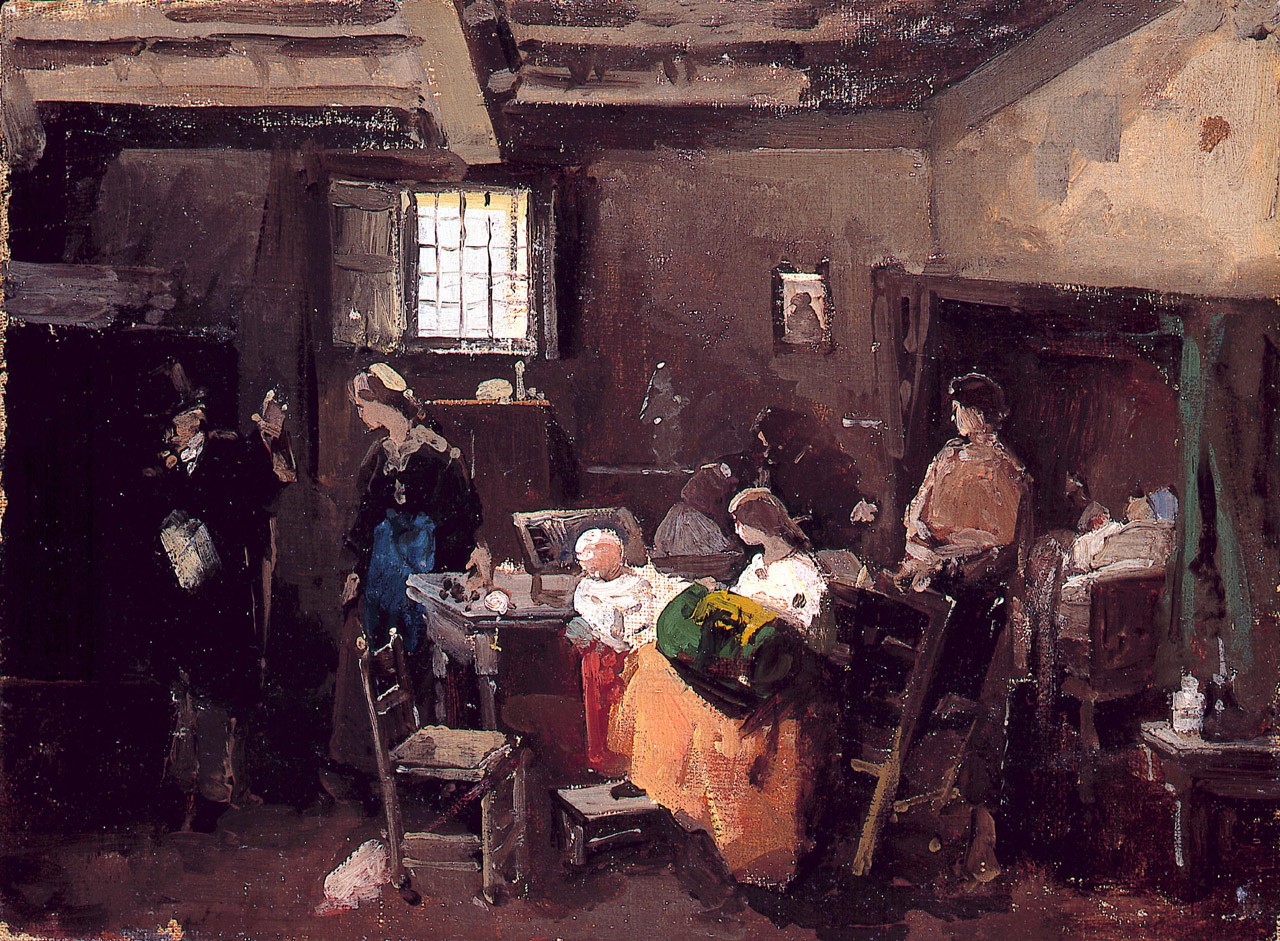This evocative oil painting, rendered in a splotchy impressionistic style, portrays a dimly lit interior of what seems to be a 19th-century cabin or house, with medium to dark brown tones dominating the room. At the heart of the scene is a brown table surrounded by various figures. A woman garbed in an orange dress sits at the table, holding a green bag with her foot resting on a stool. To her right stands a woman in a black or brown jacket with a blue apron, gazing towards a man positioned in the very left-hand corner. The man, barely visible, wears a top hat and a black jacket, with his left hand raised and possibly holding something white, like a shirt or a splotch of paint. Meanwhile, to the left of the seated woman, another woman stands with her back slightly turned, dressed in a black shirt with a white collar, a white hat, and a blue skirt. Another figure, a man in a brown shirt, can be seen standing in the background, looking down. The room also features various pieces of furniture, including a table in the far right bottom corner with a couple of jars on it and a passageway leading to what appears to be a bedroom where a figure lies down. A window with an open wooden pane brightens the upper part of the scene with a touch of yellow light, completing this atmospheric depiction of a moment frozen in time within an old-style building.